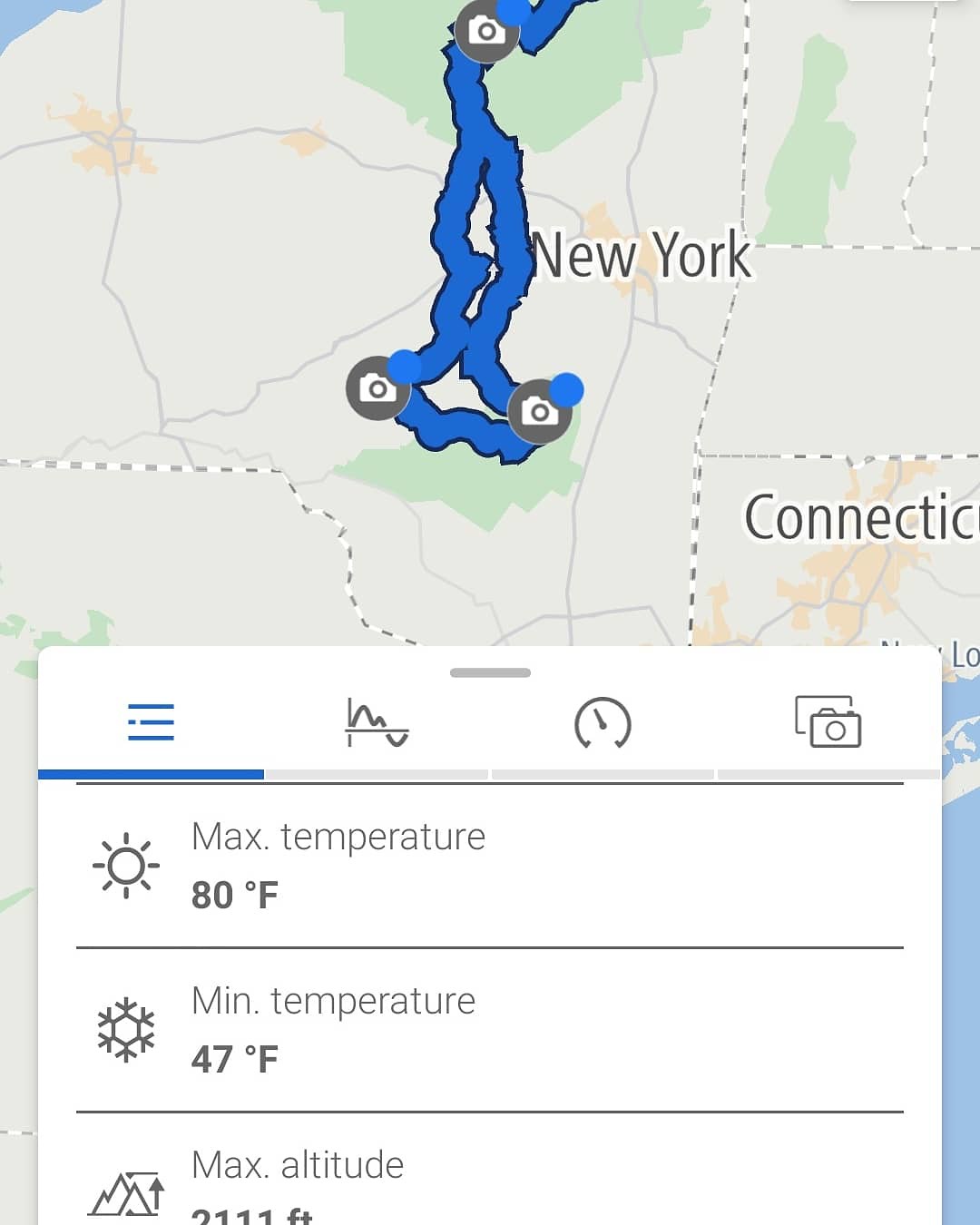This image is a detailed close-up of a digital map displaying search results primarily featuring the state of New York, with Connecticut visible to the southeast. The map showcases part of the Atlantic Ocean. Superimposed on the map is a prominent white information box providing data: the maximum temperature recorded is 80 degrees Fahrenheit, and the minimum temperature is 47 degrees Fahrenheit. Unfortunately, the maximum altitude value is partially obscured and therefore unreadable. A notable feature on the map is a blue route line connecting three unspecified locations, forming a near-loop. Despite the detailed map renderings, the specific locations along the route are not labeled, and there is no additional identifying information provided in the search results.